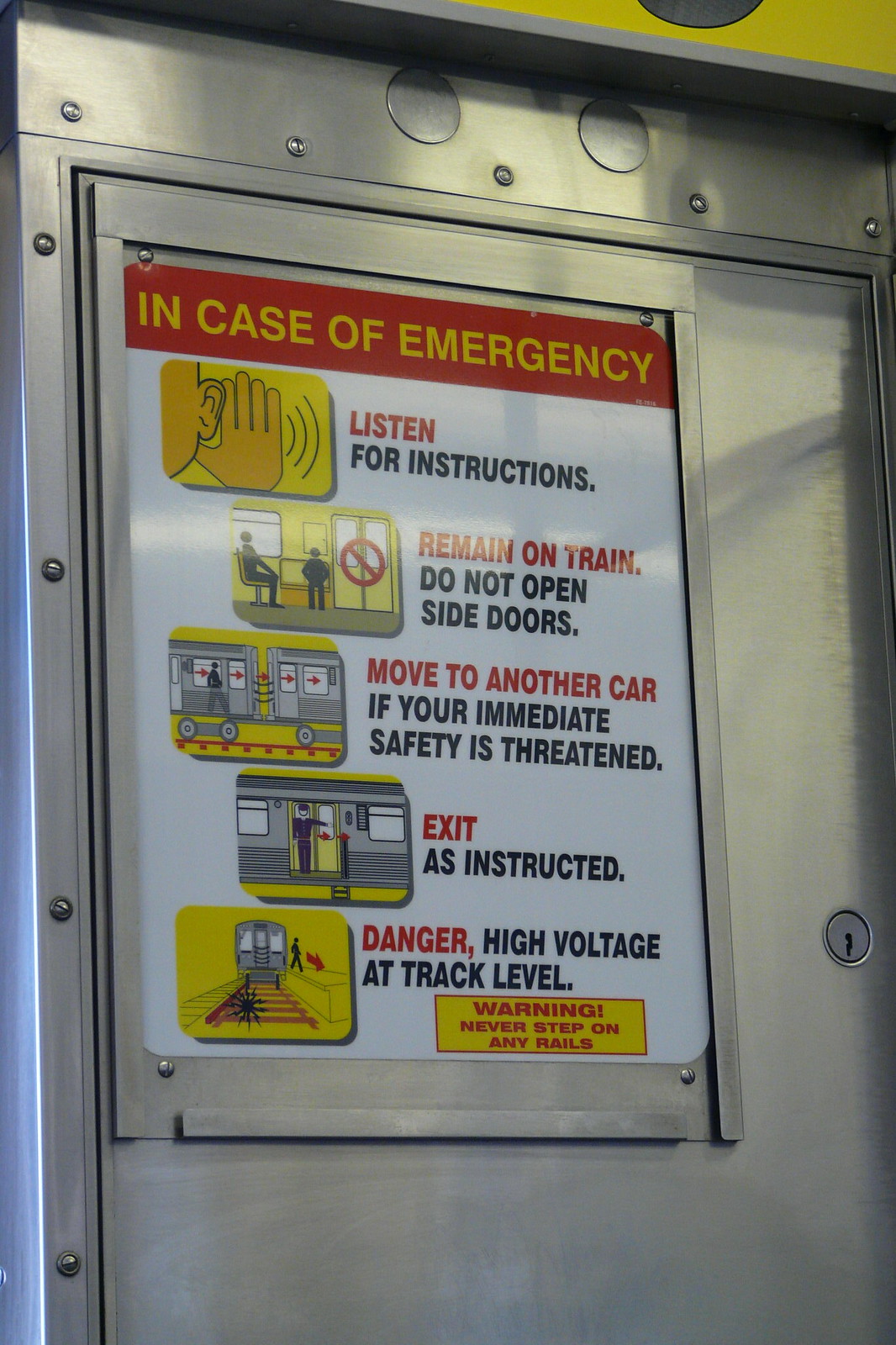This is a detailed photograph of a white plastic emergency instruction sign mounted on a silver metal panel inside a train. The metal panel features multiple small bolts and a keyhole on the right side. The sign is visually segmented with text and graphics guiding passengers on emergency procedures. At the top, a red banner with yellow lettering reads, "In Case of Emergency". Below it, an illustration of a person with a hand to their ear accompanies the directive, "Listen for Instructions." The next section advises, "Remain on Train. Do Not Open Side Doors," depicted by two seated figures and a crossed-out icon of a train door. Further down, an illustration of individuals moving between carriages is paired with the instruction, "Move to Another Car if Your Immediate Safety is Threatened." The subsequent directive, "Exit as Instructed," is illustrated with a conductor opening a door. Finally, a warning of "Danger, High Voltage at Track Level," illustrated by a person near an electrified track, cautions passengers with the statement, "Never Step on Any Rails," located at the bottom right corner of the sign.